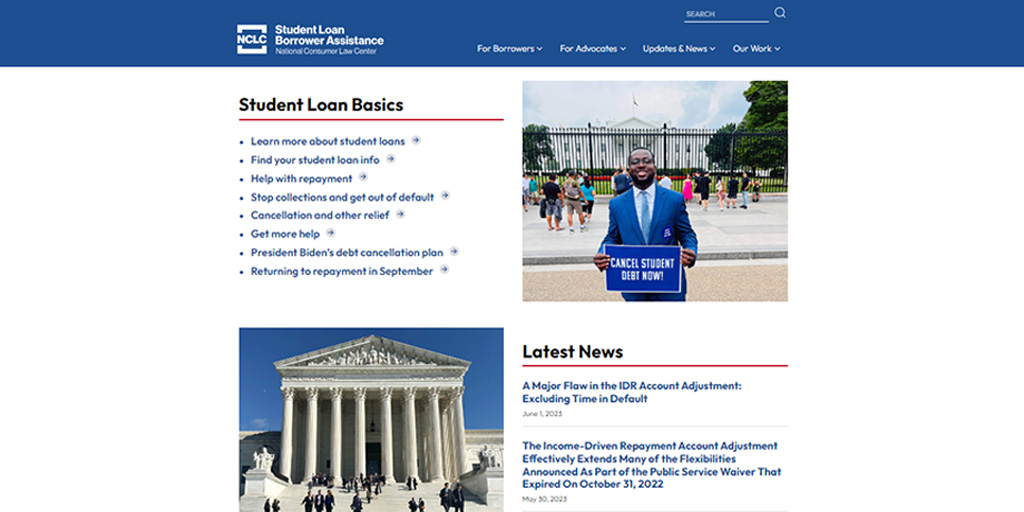This image is a screenshot from the "Student Loan Borrower Assistance" web page presented by the National Consumer Law Center (NCLC). At the top of the page, there is a blue rectangle banner displaying the text "Student Loan Borrower Assistance" alongside a boxed acronym "NCLC," which stands for National Consumer Law Center. 

To the right of this banner, there are drop-down menus with the following labels: "For Borrowers," "For Advocates," "Updates & News," and "Our Work." Below the banner, the webpage is divided into notable sections. 

The "Student Loan Basics" section is prominently featured, offering a series of clickable bullet-point links, which cover topics such as:
1. Learn More About Student Loans
2. Find Your Student Loan Info
3. Help With Repayment
4. Stop Collections and Get Out of Default
5. Cancellation and Other Relief
6. Get More Help
7. President Biden's Debt Cancellation Plan
8. Returning to Repayment in September

Adjacent to this is the "Latest News" section, which contains two articles that users can read and click on for more information.